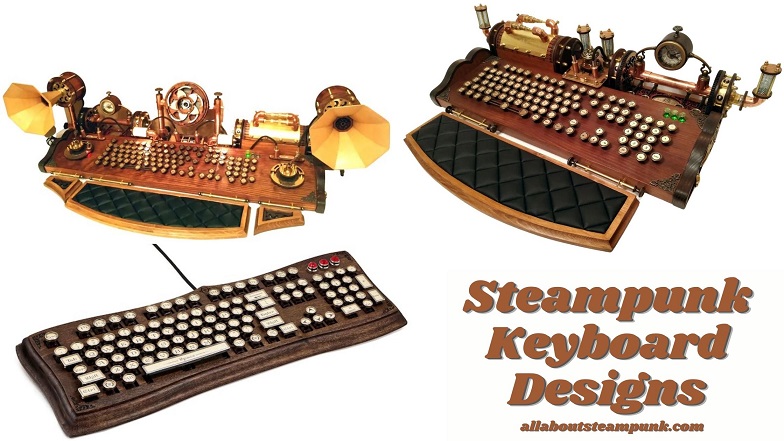The advertisement showcases three unique Steampunk Keyboards against a white background. In the bottom right-hand corner, bold, shadowed dark brown text reads "Steampunk Keyboard Designs," with the website "allaboutsteampunk.com" displayed below in a slightly smaller font. The ad features three distinct keyboard designs, each exuding a vintage, mechanical aesthetic. 

One keyboard, in the lower-left, is rectangular with a dark wood finish and round typewriter-style keys. A second, positioned in the upper left, is lighter brown and adorned with old-fashioned speakers on either side, accompanied by a central mechanical clock-like feature. In the upper right, the third keyboard stands out with its larger size, round keys, a quilted mouse pad, and telegraph-inspired instruments on top. Each keyboard is thoughtfully designed, blending historical elegance with modern functionality, and some include ergonomic hand rests for added comfort.